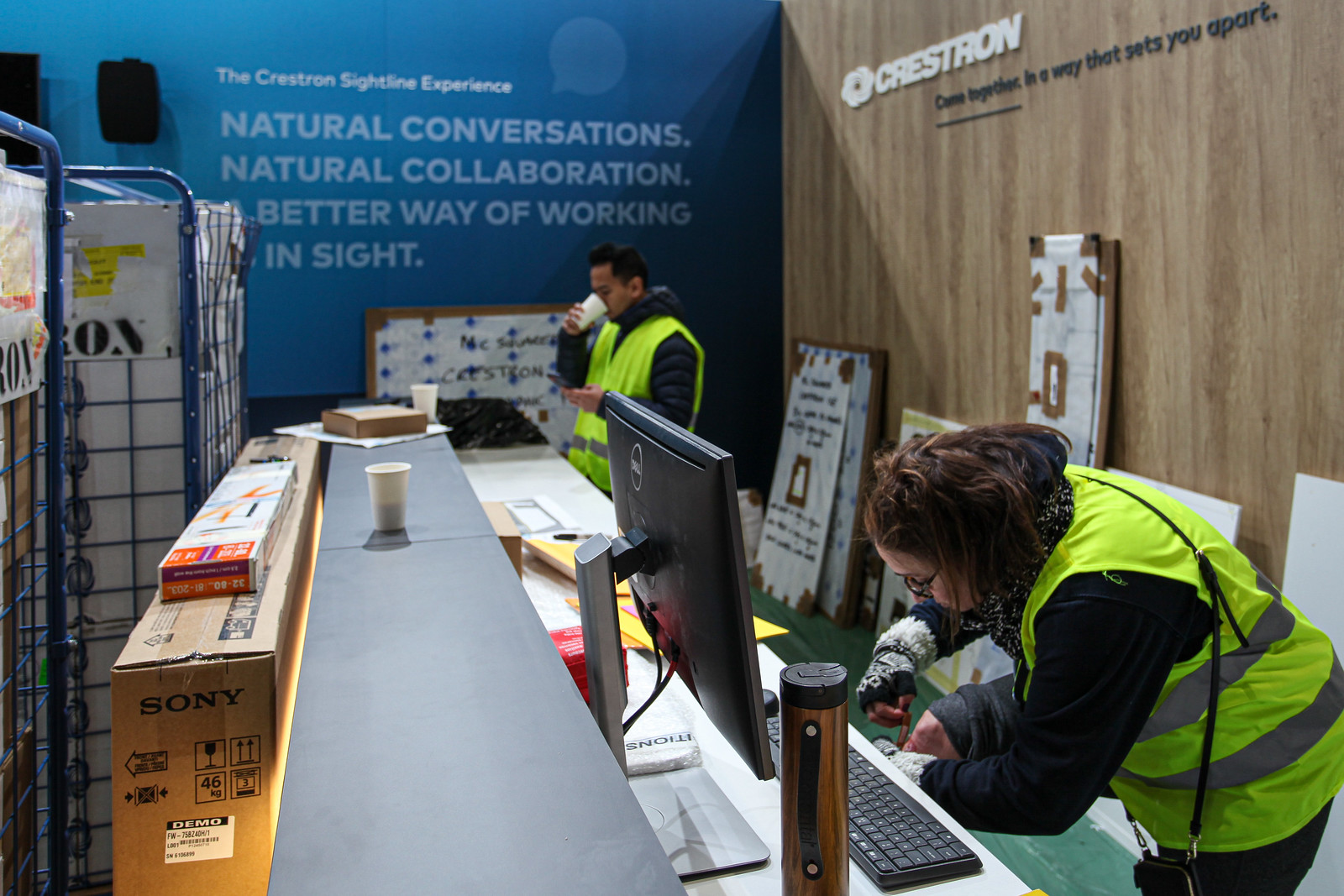The image showcases a busy scene in a tech workspace or warehouse. Two workers, both donning bright yellow vests with gray reflective stripes, are standing behind a gray counter that sits atop a white table. The female worker on the right has brown hair and is wearing a black hoodie. She is attending to her knee, possibly addressing an injury, with her knee propped up, her pants rolled up, and her fingers near her knee, which suggests she may be bandaging it. Beside her, there are papers and a thermos on the counter as she sits in front of a computer monitor with a keyboard.

Across from her, another worker with dark hair is seen drinking from a white styrofoam cup while looking at his phone. Surrounding them, the area features various storage items, including blue metal crates and a cardboard box with a Sony TV inside. To the right, a prominent brown wooden wall is displayed with the words "Crestron" written in white, followed by the slogan "Come together in a way that sets you apart" in black. In the background to the left, another blue wall bears the text "Natural conversations, natural collaboration, better way of working in sight" along with "Crestron" and "Cytron sight line experience." The setting is evidently a mix of a collaborative workspace and a storage area, emphasizing efficiency and innovation.